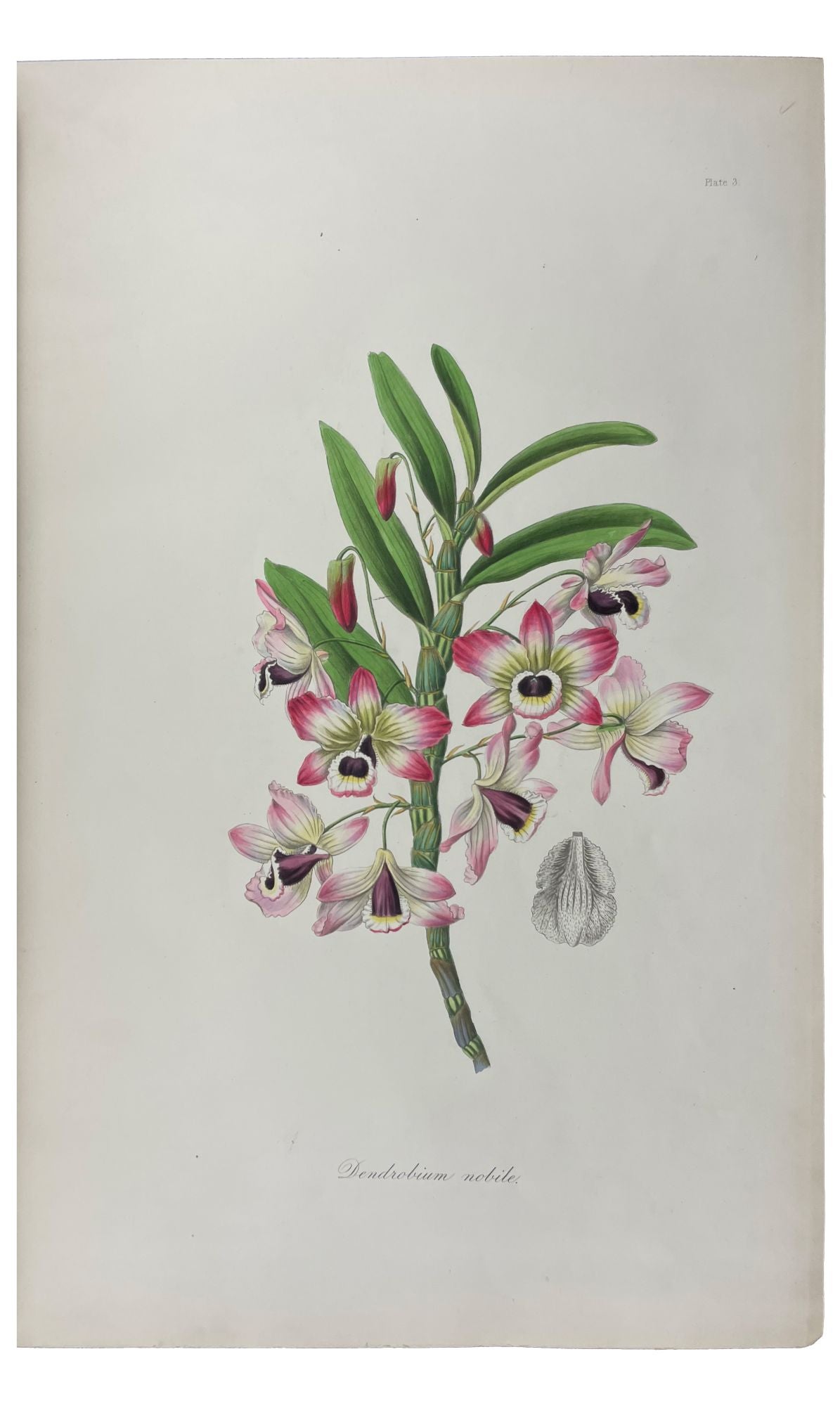The image showcases a detailed botanical illustration of what appears to be an orchid plant, specifically identified as *Dendrobium nobile*. The plant is centered on a white background, drawn or painted with precision. It features a slightly twisted and thick green stem with elongated, oval-shaped green leaves. Some flowers are in full bloom, revealing five petals each. The petals exhibit a gradient of colors with pinkish violet tips, transitioning to white towards the center, and a dark burgundy at the stamens. There are also buds that have yet to bloom, adding to the detailed depiction of different stages of growth. The background includes minimal text that is difficult to read, possibly indicating a page number and the plant's scientific name in cursive and small print. Additionally, a black-and-white drawing of the plant appears at the bottom right, providing further botanical detail.